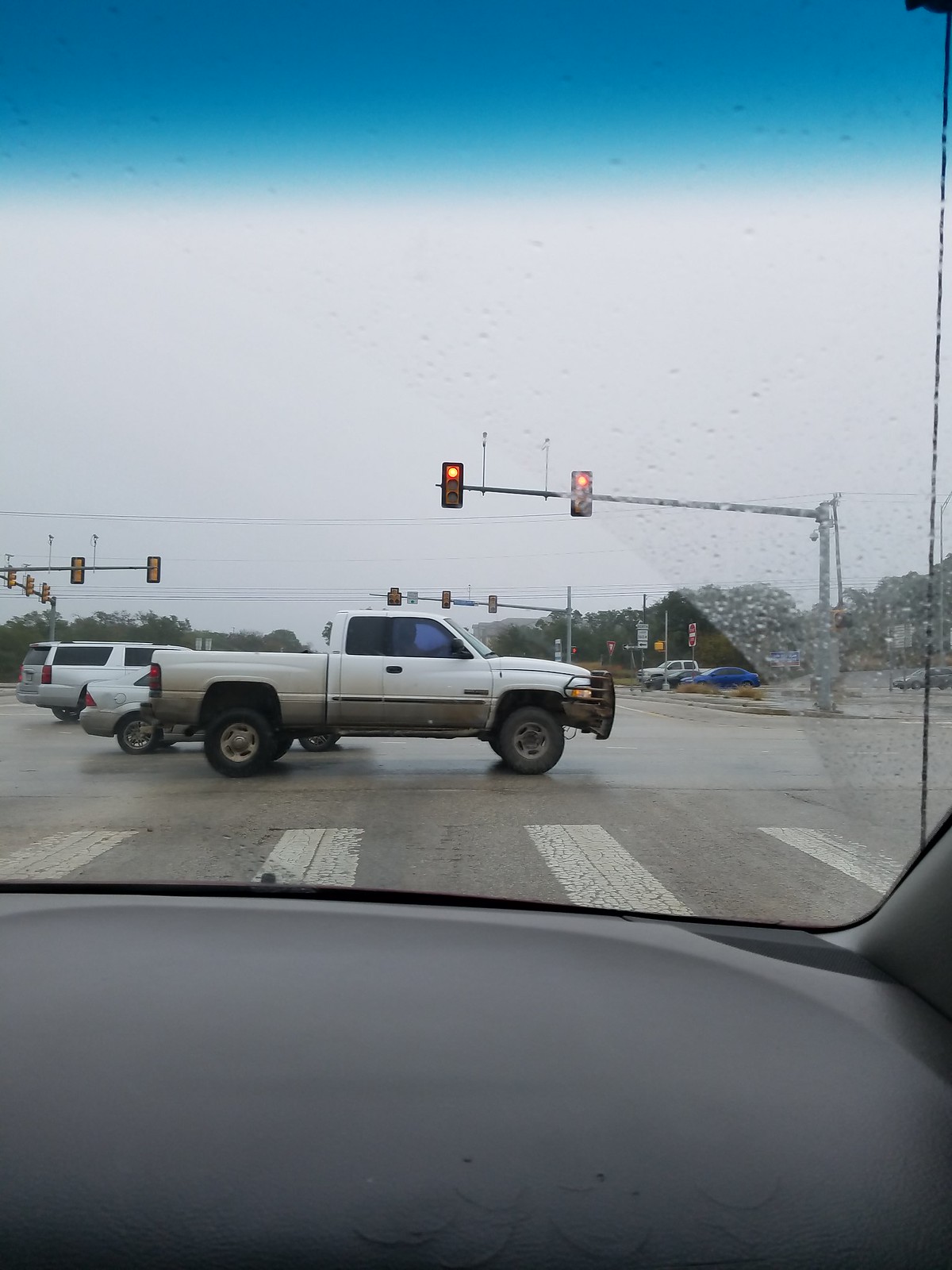The photograph is taken from inside a stationary vehicle at a red light, with the dashboard visible at the bottom. The windshield is dotted with raindrops, with clear streaks from the wipers revealing the scene beyond. The sky is a dramatic gradient, vibrant blue at the top fading into a gray, indicating overcast weather despite some brightness suggesting the sun is behind the clouds. The main focus is a white, somewhat dirty double cab pickup truck driving horizontally through a busy multi-lane intersection. Following it is a silver car and a silvery white station wagon making a left turn. Additional cars— a white truck, a black car, and a royal blue car—queue behind. Above the intersection are traffic lights, all displaying red. A "Do Not Enter" sign and some background details of a wall with gravel or dirt below add context to the urban setting.